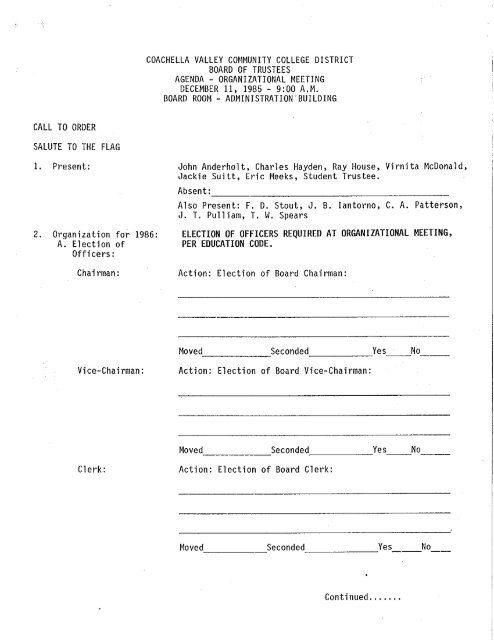This is a scanned document from the Coachella Valley Community College District, titled "Board of Trustees Agenda - Organizational Meeting, December 11, 1985, 9 a.m., Boardroom, Administration Building." It outlines the agenda, starting with "Call to Order" and "Salute to the Flag," then lists attendees: John Anderholt, Charles Hayden, Ray House, Vernita McDonald, Jackie Soltz, Eric Meeks, and a Student Trustee with none absent. Other attendees include F.D. Stout, J.B. Iantorno, C.A. Patterson, J.T. Pulliam, and T.W. Spears. The document features fill-in-the-blank sections to record elections for Chairman, Vice Chairman, and Clerk, as required by the education code. It also includes spaces to write the actions taken, such as who moved and seconded motions, and the results of votes. The detailed layout of the form includes areas to note ongoing business indicated by "continue......" at the bottom.